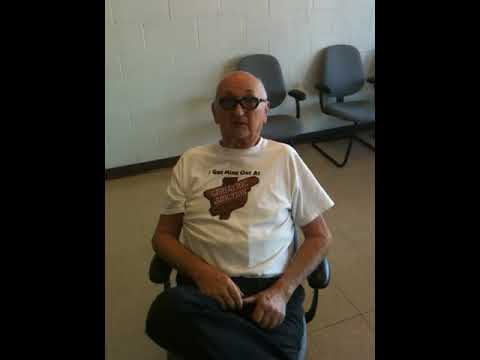This photograph captures an elderly Caucasian man, likely in his late 60s or 70s, seated in a low-backed, office-style armchair with black framing. He wears thick-rimmed glasses and sports a bald head. His attire includes a light-colored, short-sleeve t-shirt, adorned with a cartoonish wooden diagonal road sign featuring unreadable text in its center, and additional small black lettering above it. He pairs this with indistinguishable dark pants, either trousers or jeans. The gentleman's right leg is crossed over his left thigh, and his arms are bent at the elbows, with his forearms resting on the armrests of the chair and his hands in his lap. He gazes directly into the camera, maintaining a neutral expression. The setting appears to be a waiting room with a white wall, a black baseboard, and a light tan or wood floor. Behind him, two similar gray office-style or waiting room chairs with black metal legs are aligned against the wall. The photo is bordered on the left and right by two vertically aligned, rectangular black panels.